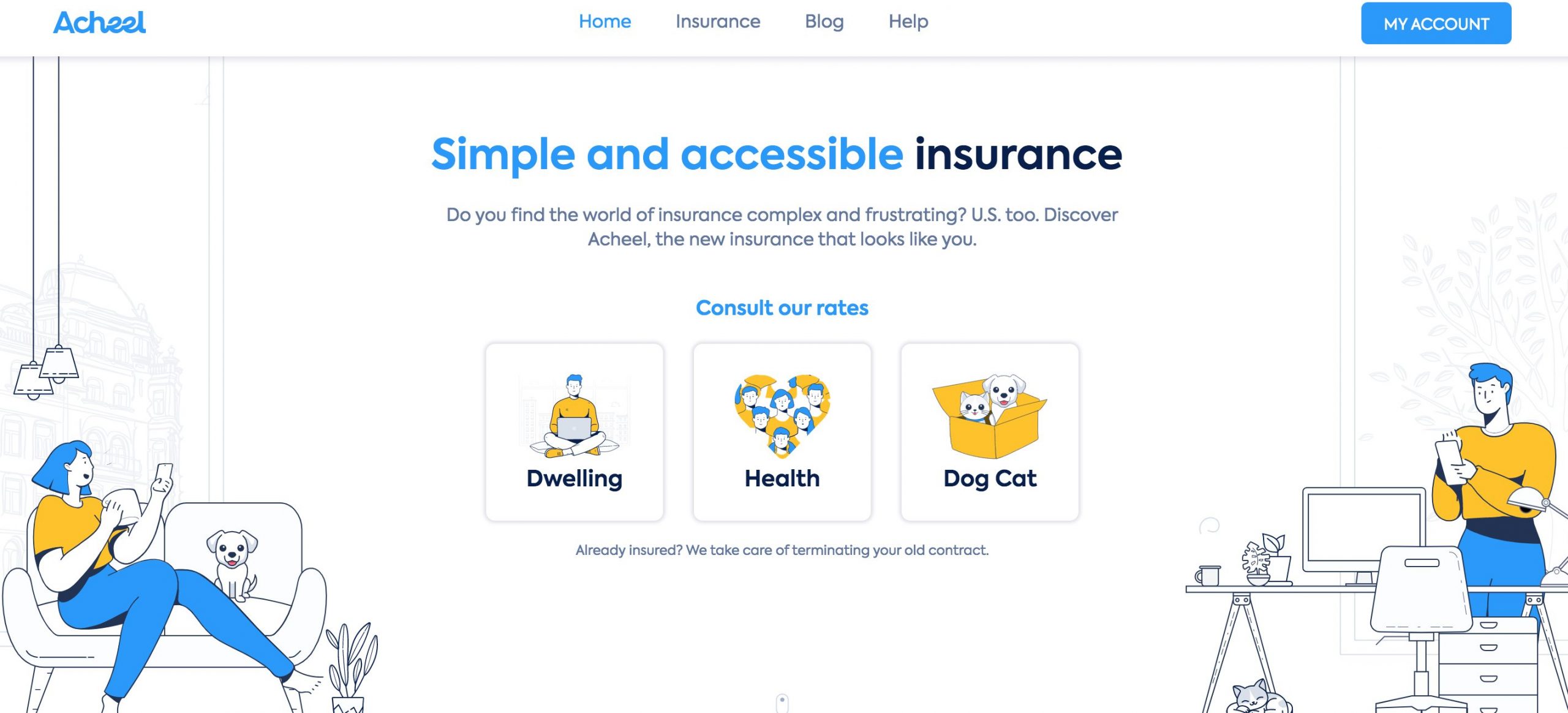The image depicts the homepage of a company called ACH EEL, prominently showcasing the tagline "Simple and Accessible Insurance." The ACH EEL logo is positioned in light blue in the upper left-hand corner. The navigation bar at the top features "Home" highlighted in blue, while "Insurance," "Blog," and "Help" are displayed in black. A blue box in the upper right-hand corner labeled "My Account" invites users to click.

Below the tagline, written in light blue for "simple and accessible" and black for "insurance," is a welcoming message that reads: "Do you find the world of insurance complex and frustrating? Us too. Discover ACH EEL, the new insurance that looks like you." The site features icons representing various services: dwelling, health, and pet insurance (dog and cat).

In the lower left-hand corner, a woman with blue hair, wearing blue pants and an orange shirt, sits on a couch. She appears to be looking at her phone or talking on it, with a dog sitting beside her. A plant can be seen next to her leg.

In the lower right-hand corner, a man with blue hair, also dressed in blue pants and an orange shirt, is seated at a desk. He seems to be working on something, with a computer on the desk, and a plant nearby. A cat is sleeping beneath the desk, adding a cozy touch to the scene. The desk chair is also visible in this detailed and engaging depiction of ACH EEL’s approachable and user-friendly insurance services.